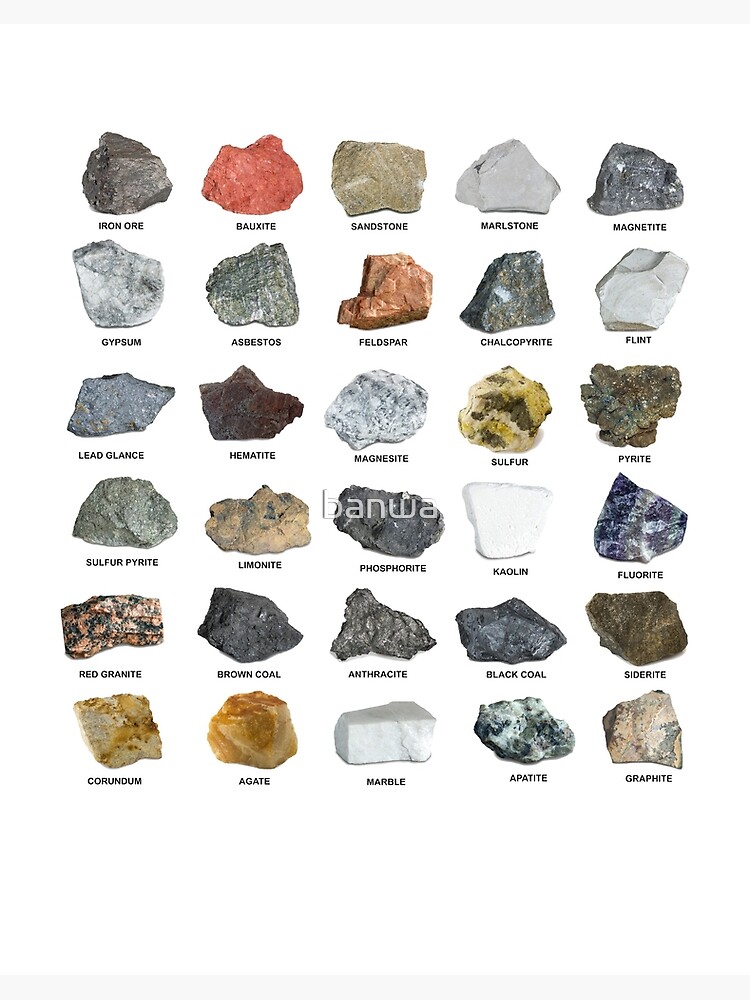The image displays a detailed rock collection, meticulously arranged on a white background. The collection features 30 different types of rocks, laid out in a grid of five columns and six rows. Each rock is affixed and identified with a small, readable label beneath it, listing names such as iron ore, bauxite, sandstone, milestone, magnetite, gypsum, asbestos, feldspar, chalcopyrite, hematite, red granite, magnesite, agate, marble, black coal, and blue fluorite. The rocks showcase a variety of colors, including tans, silvers, grays, browns, reds, corals, amber golds, and blues, highlighting the natural variations and layered formations of each specimen. The rocks range in texture from rough to uneven, emphasizing their unpolished, natural states. Lightly printed in the middle of the collection is the word "BANWA," suggestive of the company or organization associated with this impressive display. The combination of vivid colors, varied textures, and precise labeling make this an educational and visually captivating collection for rock and mineral enthusiasts.